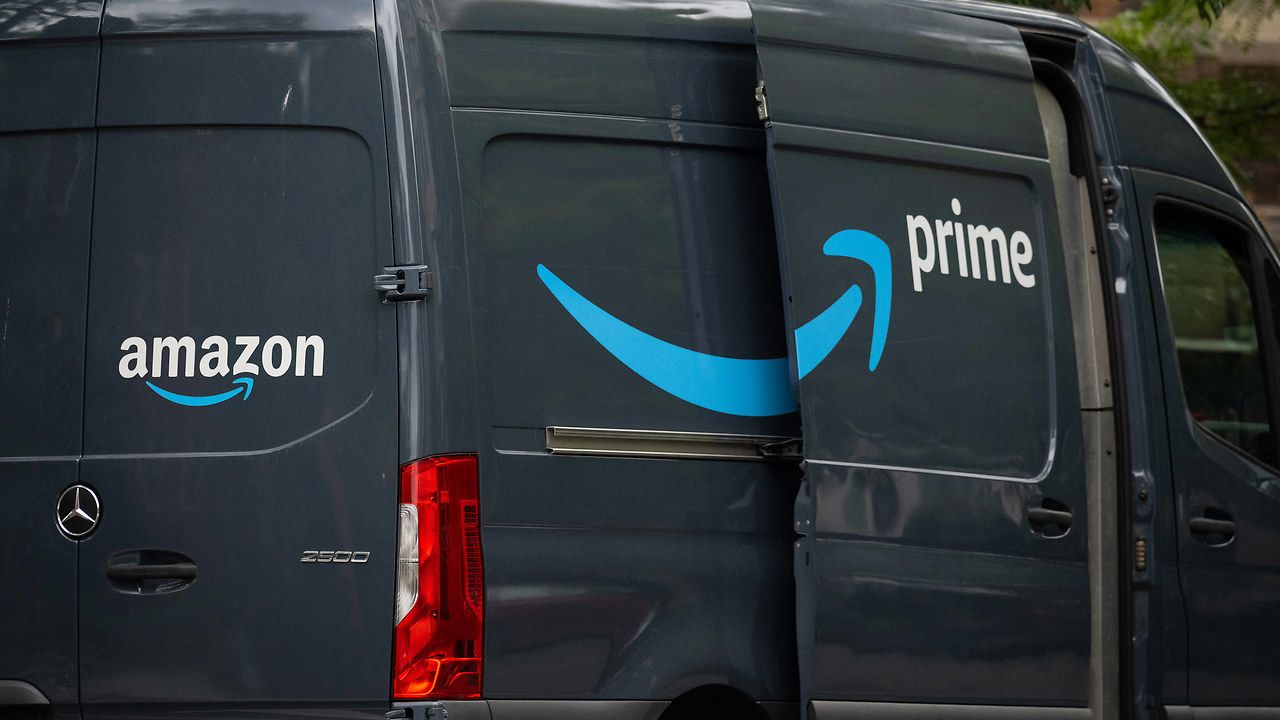In the image, a dark gray Amazon Prime delivery van, specifically a Mercedes 2500 model, is prominently featured. The van's side sliding door is open, revealing the vehicle's interior, and it has two hinged doors at the rear, which are also slightly ajar. The distinct Amazon Prime branding is visible; the blue, curved arrow logo is displayed prominently along with the "Prime" text in white font on the side, and the word "Amazon" with the same blue arrow is placed at the rear. The Mercedes emblem, a silver circle with a three-pointed star, is noticeable at the front of the vehicle, accompanied by the number "2500" near the black door handle. The scene is set in a residential area, with glimpses of trees and the brick exterior of a house providing a backdrop to the parked van.